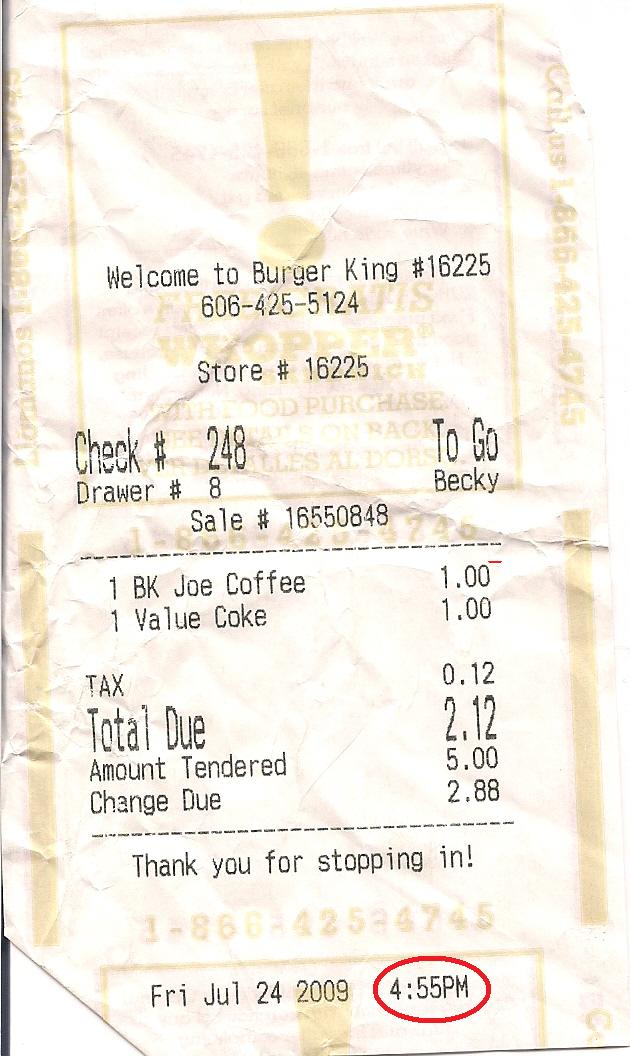A crinkled off-white receipt from Burger King is shown, appearing well-worn as if it had been folded and kept in someone's pocket. The header reads "Welcome to Burger King," identifying the customer as number 16,225. The receipt, dated Friday, July 24, 2009, at 4:55 p.m. (with the time prominently circled in red), details the purchase of one black coffee for $1.00 and a small Coke for $2.00. The subtotal before tax is $2.00, with an additional twelve cents in tax, bringing the total amount due to $2.88. Additionally, the cashier's name, Becky, and the drawer number, eight, are indicated on the receipt. The telephone number of the establishment is also provided.